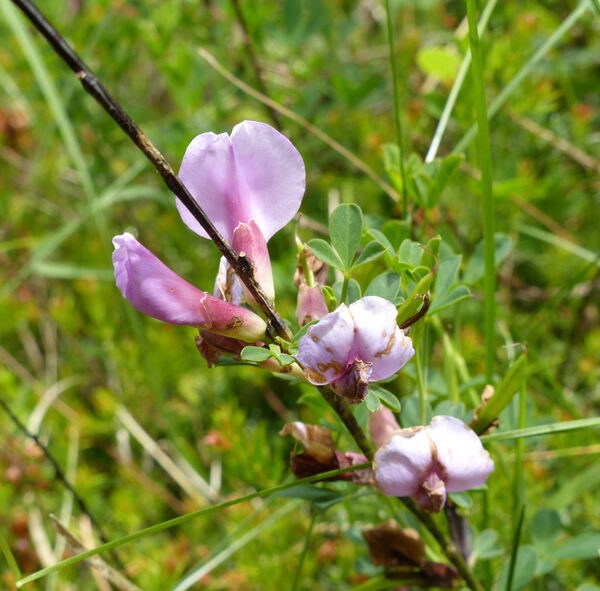In this detailed nature photograph, the focus is on a purplish-pink wildflower situated on a thin, brownish branch with green leaves. The flower, which appears to be in poor condition, shows signs of withering with some brown patches on the petals. The branch stretches diagonally across the image from the top left, making it the main element in focus. Behind the flower, there is a backdrop of tall, green grasses, various other wildflowers, and weeds, indicative of an outdoor wilderness setting, likely during spring or summer. The image captures a range of earth tones including browns, greens, and shades of pink, emphasizing the colorful yet natural setting. The background is blurred, highlighting the detailed texture and color of the flower in the foreground. The photograph contains no text and radiates a natural, untouched aesthetic of a secluded outdoor area.